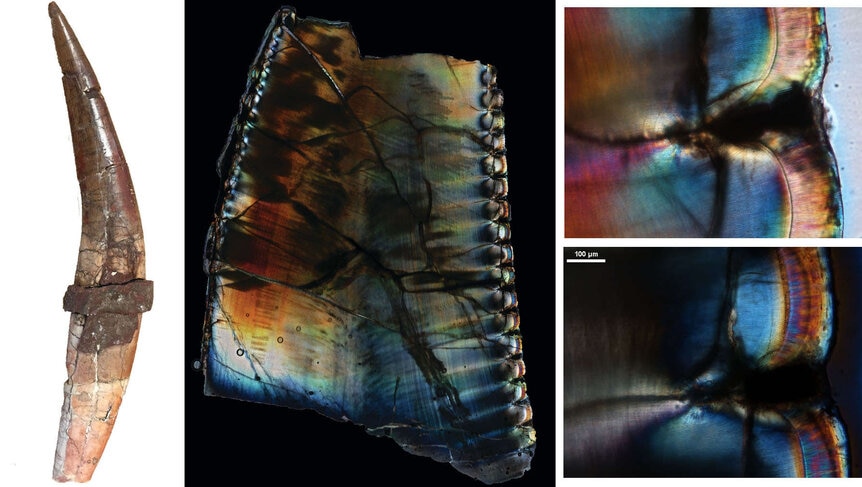The image comprises four distinct photos centered around what appears to be a large, fossilized tooth. The main photo on the far left shows the tooth against a white background, resembling a curved dagger. The tooth features a gradient coloration: it is whiter on the bottom and transitions to a brown hue towards the top, with its pointed tip angled towards the upper left corner. To the right of this image, there are three additional microscopic close-ups of the tooth, displaying extensive detail such as small cracks and intricate striations. These microscopic images are color-enhanced, showcasing shades of blues, yellows, and greens, likely achieved using specialized lighting techniques. The three secondary photos include one nearly full-tooth close-up in the center left, and two highly magnified sections on the far right, revealing more intricate details and some labelled measurement, indicating "100 UM."